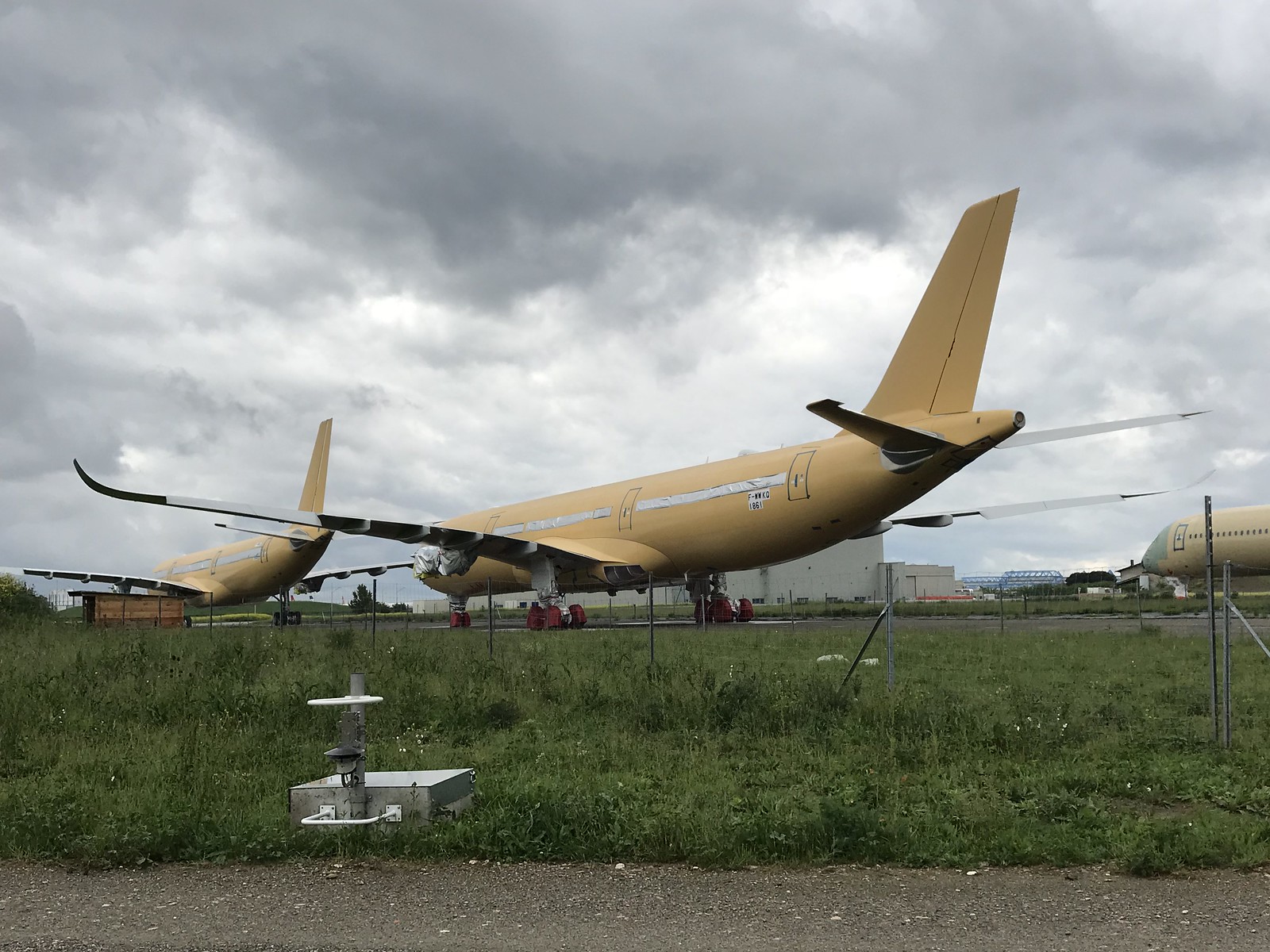The image depicts a cloudy, possibly pre-rainy day at an aircraft storage or maintenance area, featuring three beige commercial jets. In the foreground, there is a gray gravel road, a grassy expanse, and a chain-link fence. Behind the fence, the jets are parked with their noses pointing slightly to the left of the image. The closest jet is centrally located, with another to its left and the nose of a third jet visible on the right. Each jet has a white strip along where the windows would be, and their left wings are prominently visible. The tires of the jets appear red. In the background, several structures, possibly hangars, are visible under ominously dark clouds. Additionally, there is a silver box with a spigot at the base of the grass near the fence. The overall scene suggests the aircraft might be undergoing repairs, used for parts, or potentially kept for training purposes.